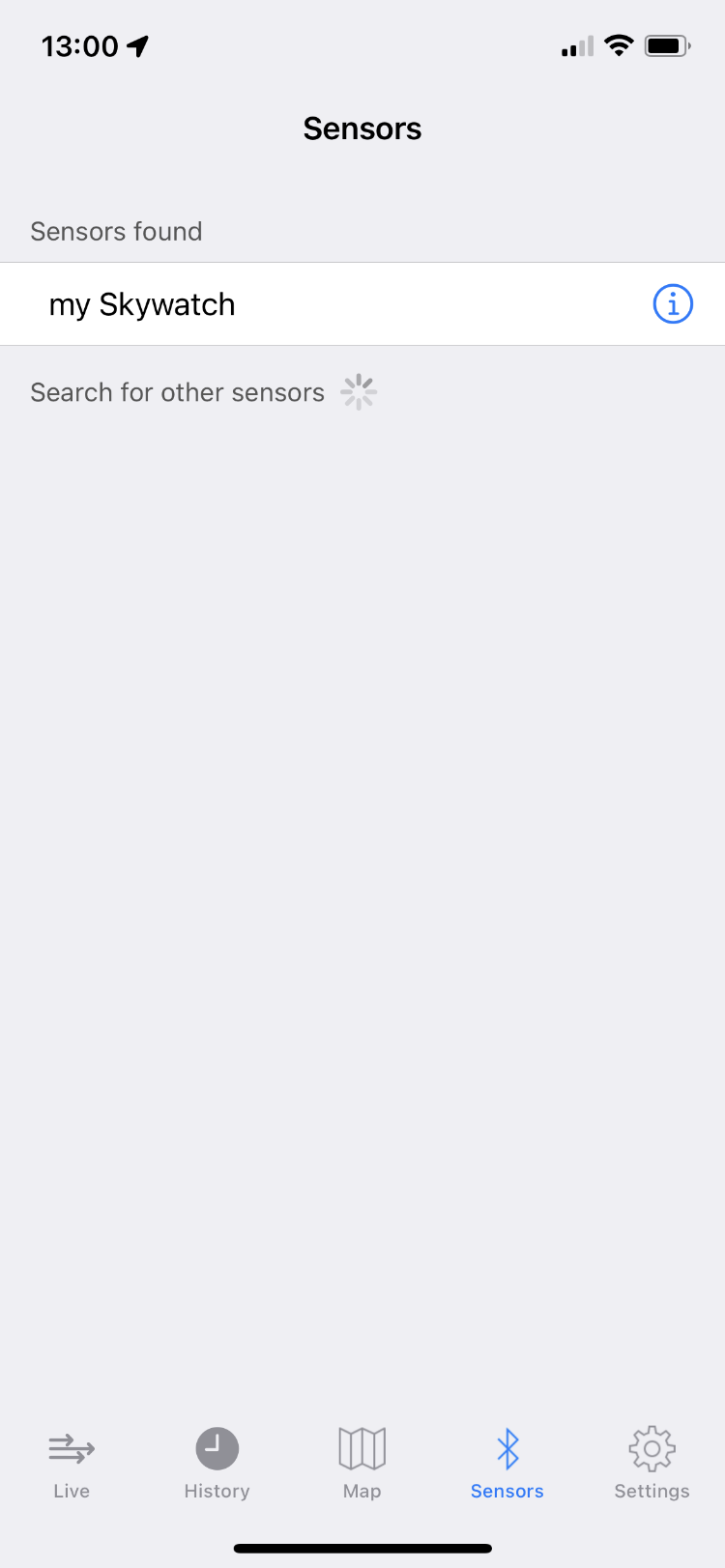The image is a screenshot from a smartphone, featuring a minimalist and functional user interface on a pale gray background. Dominating the upper portion of the screen is a thin, horizontal, white rectangular box that contains the text "my Skywatch" in a blend of lowercase and uppercase letters, with "my" in lowercase and "Skywatch" starting with an uppercase "S." The text is printed in black lettering. Above this box, the phrase "sensors found" is displayed, while directly below it is the prompt "search for other sensors."

To the right of the "Skywatch" text within the white box, there is a blue circle that encloses a lowercase "i," signifying an information icon. In the upper-left corner of the screen, the military time "13:00" is visible, accompanied by an upward and rightward-pointing locator arrow. Opposite this, in the upper-right corner, standard status indicators for Wi-Fi, battery, and cell signal strength are present. 

At the bottom of the screen, a series of icons are arranged in a horizontal row, each paired with a descriptive label. The icons and their corresponding functionalities from left to right are:
1. "Live," accompanied by right-pointing arrows.
2. "History."
3. "Map."
4. "Sensors."
5. "Settings."

Each of these icons includes distinct symbols positioned above the text to visually represent their functions.